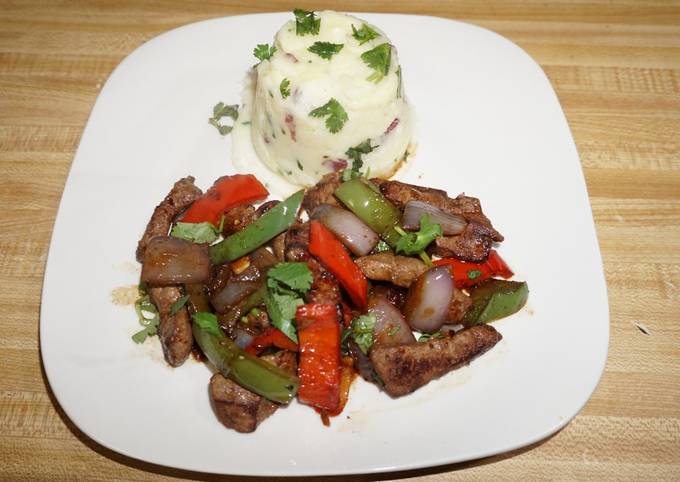The image displays a tantalizing meal presented on a large, square white plate with rounded corners, placed on a light pine wood table, showcasing the grain of the wood. At the top of the plate, there's a mound of mashed potatoes, mashed with the skins on, revealing flecks of red skin throughout. The mashed potatoes are garnished with chives and possibly other herbs. Adjacent to the potatoes is a generous portion of stir-fried peppered steak, featuring succulent strips of brown beef, intermixed with sautéed green and red bell peppers, onions, and garnished with cilantro. The stir-fry has a shiny, slightly greasy appearance, indicating a savory sauce that coats the ingredients. The composition of the meal, vibrant and visually appealing, sits against a backdrop reminiscent of a butcher block, adding to the rustic charm.